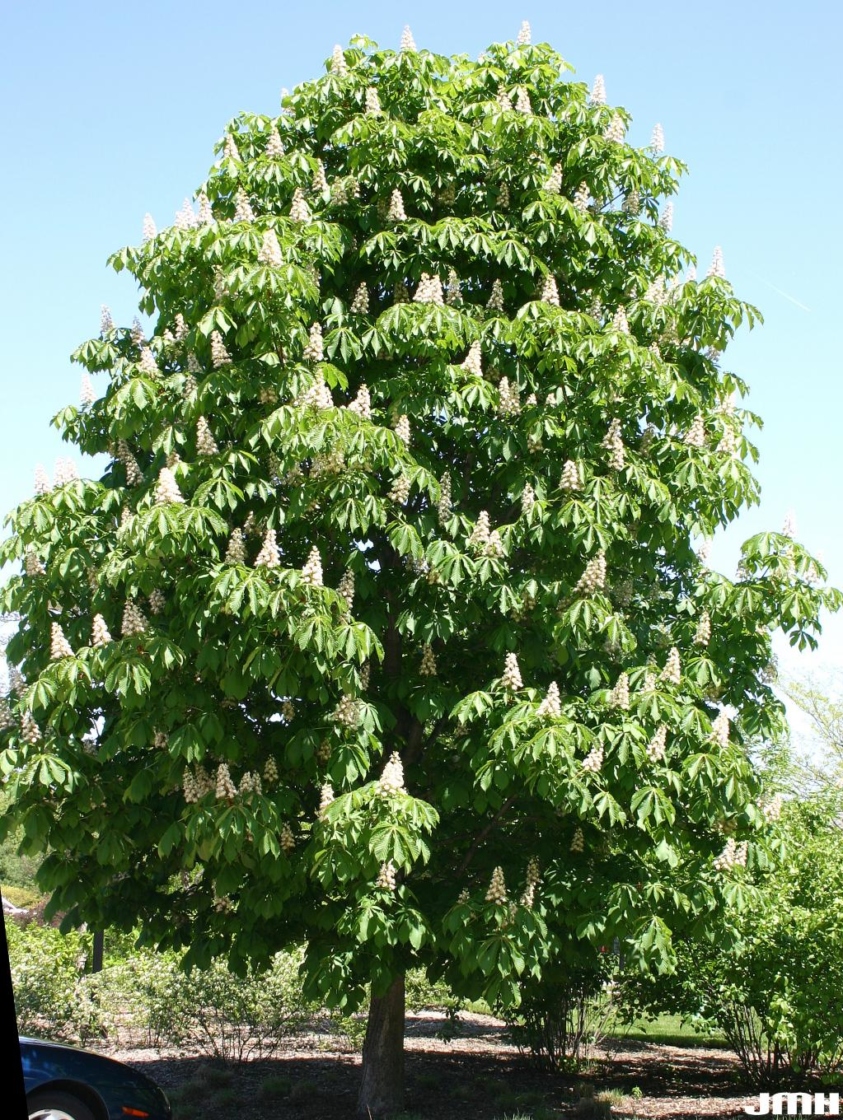This image prominently features a very large and tall flowering tree in full bloom, set against a completely clear, blue sky with sunlight streaming down. The tree's thick foliage comprises clusters of green leaves interspersed with white flowering clusters that resemble tiny Christmas trees. The trunk of the tree is long and sturdy, and it gives the appearance of a mature, healthy tree thriving in what seems to be a spring setting. 

On the right side of the tree, there is a bush, and the ground around the tree is mainly brown dirt, dotted with some low shrubs. There are shadows cast over parts of the dirt, but sunlight filters through in places, creating a patchwork of light and shadow on the ground. In the bottom right-hand corner of the image, the initials "J-M-H" are visible, presumably signifying the photographer. Additionally, on the bottom left side, part of a parked car with a dark black color is visible, specifically the front section and part of the front wheel. This comprehensive scene captures a peaceful, sunlit moment with the flowering tree as its central focus.